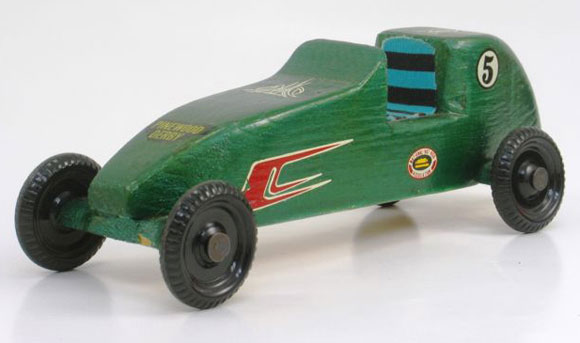This close-up photograph depicts a handcrafted Pinewood Derby car, styled as a rudimentary race car, set against a white background. The car's body, made from a block of wood, is painted a dark green, almost entirely covering its surface. It features four black wheels, though only three are visible in the image. Prominently displayed on its side is a black number 5 within a white circle. Just behind the number 5, a red flame design, outlined in white and shaped like a pointy "C," adds a dynamic touch. The vehicle's cockpit area, where a toy driver would sit, is marked by a seat painted with blue and black stripes. Various decals adorn the car, including an unreadable sticker with a black background and yellow lettering on top, and an intricate white tribal symbol situated on the hood. An additional circle emblem with indistinct details is positioned beneath the seat.